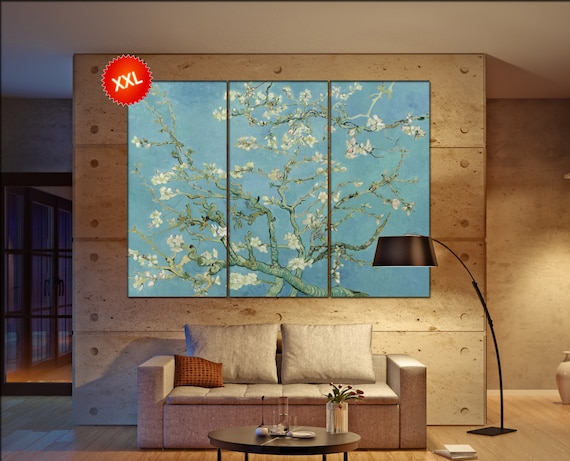In this indoor nighttime photograph, a cozy living room or lobby is depicted with a variety of elegant and oriental-inspired accents. The focal point is a two-seat grey sofa, also known as a love seat, adorned with two grey pillows and a smaller orange pillow on the left side. Positioned in front of the sofa is an oval-shaped coffee table, which holds a rectangular vase filled with vibrant red flowers, thin glass vases, and an assortment of glasses. 

A striking floor lamp with a black shade arches gracefully to the right of the sofa. The backdrop features a warm wooden wall on which hangs a triptych painting of a tree adorned with white blossoms, aligned across three panels. Adding to the room's Japanese feel, there is a sense of minimalism and functional design, accentuated by the clean lines and sparse but thoughtfully placed decor.

To the right of the scene, another wall continues into the background, showcasing a white, off-white floor vase. Enhancing the wooden elements, the floor is a rich hardwood. On the left side of the image, there is a door opening into a hallway with additional doors. A red sticker-like mark in the top left corner reads "XXL," suggesting this image may be part of an advertisement. The scene is completed with a sense of tranquility and aesthetic balance, reminiscent of Japanese-style interiors.